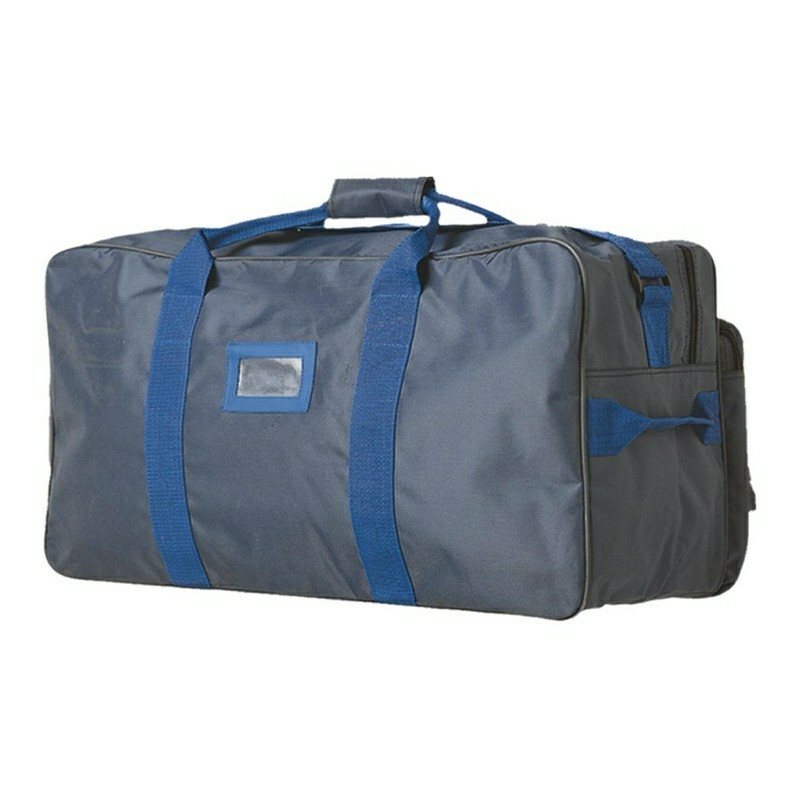This image features a basic stock photo of a grayish blue, rectangular duffel bag set against a completely white background. The duffel bag appears to be made of a canvas or nylon-style material and features various blue straps, with a truer blue for the handles and side straps. Notably, the bag has two vertical straps on its side and a top clasp that secures these handles together, matching the main bluish-gray color of the bag. On the wide side of the bag, there's a rectangular pocket bordered in blue with a clear middle section designed for a label or name tag. Additionally, there's a horizontal blue strap on the side of the bag, as well as a vertical strap. The bag appears to be zipped up and fully packed. It's described as looking somewhat old, beat up, and dirty, adding a worn, shabby appearance to the overall image.